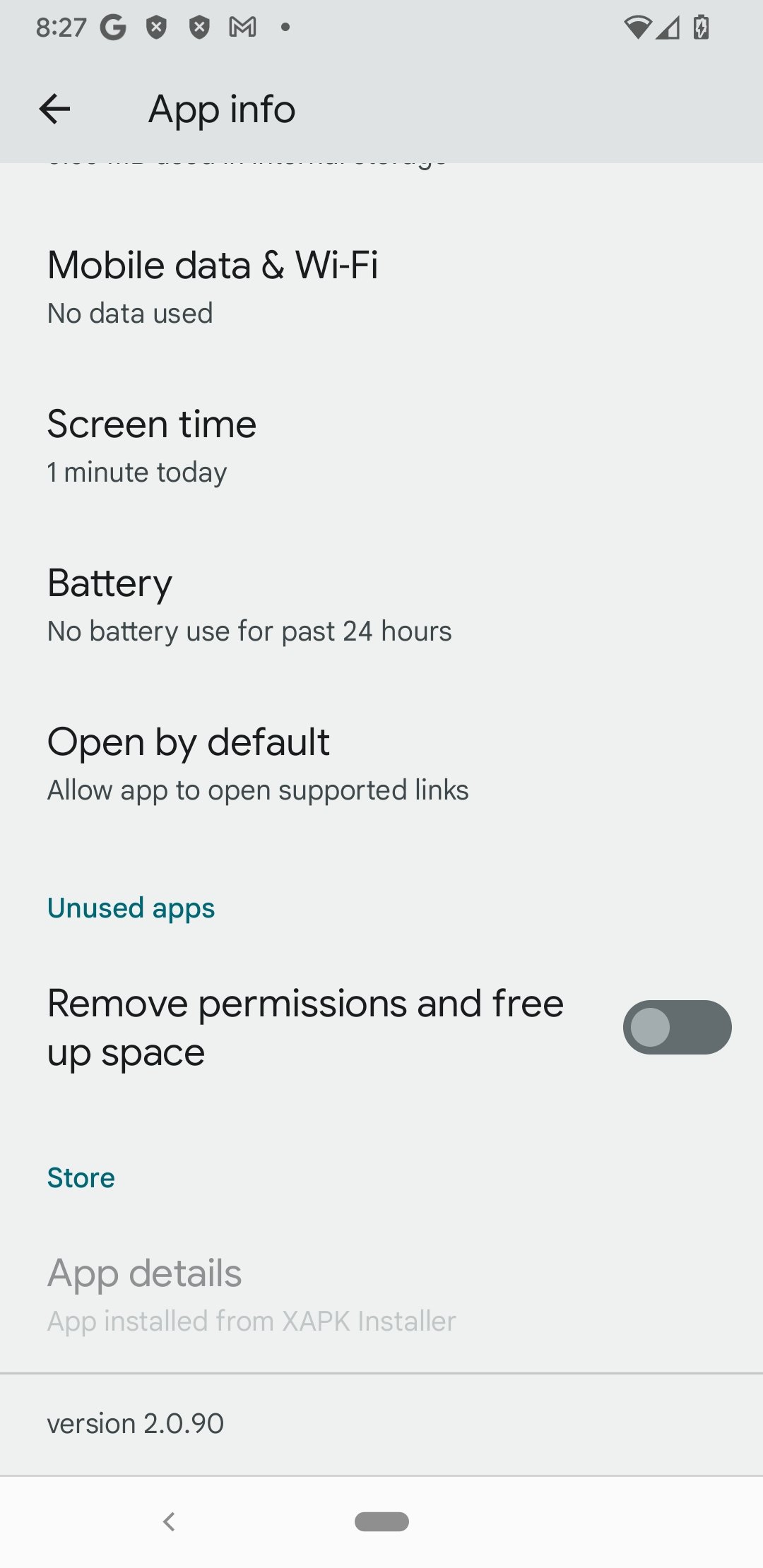The image showcases the screen of a cell phone displaying the "App Info" page for a specific application. 

At the top of the screen, there's a darker gray strip compared to the lighter gray background below it. On the left side of this strip, it displays '820', followed by a 'G', two shields with X's, an 'M', and a dot. On the right side, there are icons indicating Wi-Fi signal strength, cellular network bars, and a charging battery status.

Below, there's a left arrow icon next to the text "App info" on the lighter gray background. The main content is displayed in a list format with a black font, left-justified. Here are the detailed entries:

- **Mobile data and Wi-Fi**: States "No data use."
- **Screen time**: Shows "One minute today."
- **Battery**: Indicates "No battery use for the past 24 hours."
- **Open by default**: Allows the app to open supported links.
- **Unused apps**: Highlighted in green or teal.

Further down, there's an option to "Remove permissions and free up space," which is gray, implying it may not be toggled on. It is followed by the word "Store" highlighted in teal.

At the lower section, it specifies "App details," revealing the app was installed from "XAPK installer." Below a separating line, it mentions "Version 2.0.90".

Finally, at the bottom of the screen, navigation options appear for the phone, including a left arrow and a centrally positioned black bar.

The predominant colors on this screen include two shades of gray, black, teal, and white.